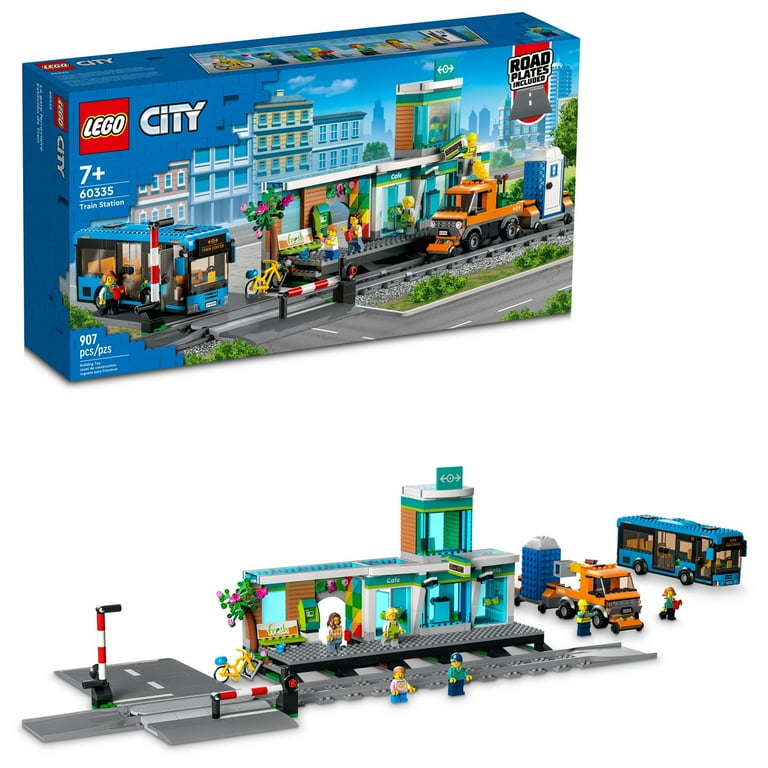The image consists of two color photographs set against a white background, showcasing a Lego City set. The top photograph displays the unopened Lego City box, which prominently features blue borders and the Lego logo in red, yellow, and white. The box is labeled 7+ and contains 907 pieces, including road plates. The depicted set features a cityscape with a rail station, a streetcar, and various accessories like a blue bus, bicycle, and a railway crossing. The bottom photograph shows the fully assembled Lego City set, highlighting a bustling street scene with six Lego figures. The setup includes a blue bus, a blue porta potty, a train depot with people waiting beside the tracks, and a small truck hauling the porta potty. This completed display brings the vibrant cityscape to life, emphasizing its dynamic elements and detailed components.